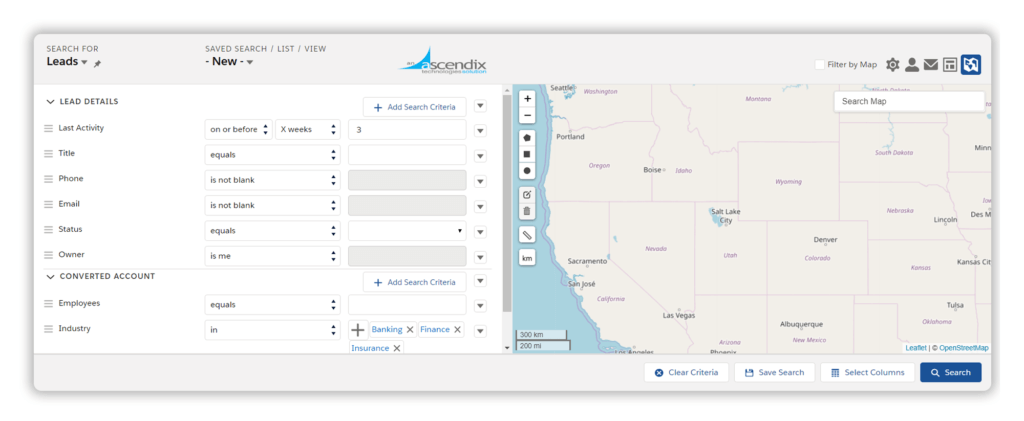The image features a light grey background with various elements arranged across it in a structured layout. 

- In the top-left corner, there is some grey writing above black text. Below this text, there's a logo featuring a blue swoosh, black letters, and additional blue letters underneath.
- On the right hand side, a series of words are accompanied by several icons: a gear, a person symbol, an envelope, a square with lines, and a blue square with some white details that are not clearly discernible.
- Beneath these icons, on the left hand side, there is a white vertical rectangle containing symbols with words next to them, although the words are not legible.
- To the right of this white rectangle, there are two grey outlined rectangles, each containing words and a symbol. Below these, there are four more similar grey outlined rectangles, each longer and similarly containing words and symbols, making a total of six.
- Further down, there is a grey outlined rectangle featuring a plus sign and some blue text, followed by another grey outlined rectangle with either a letter or number, and another blank rectangle.
- Next to these rectangles is a series of grey rectangles, one of which has some indiscernible elements on its right side. These are followed by more grey outlined rectangles, one featuring a plus sign with blue text, and another series featuring a plus sign, a blue text, and an X, repeating several times.
- The far-right side of the image exhibits a vertical row of arrows, indicating navigation or movement.
- On the left, adjacent to the map, there are three white rectangles, each containing a symbol and blue text. A blue rectangle with a magnifying glass icon and the word "Search" completes this section.

Overall, the layout is highly structured with numerous icons, symbols, and text boxes, aiming to provide a comprehensive visual guide or interface, though some text and details remain unclear.